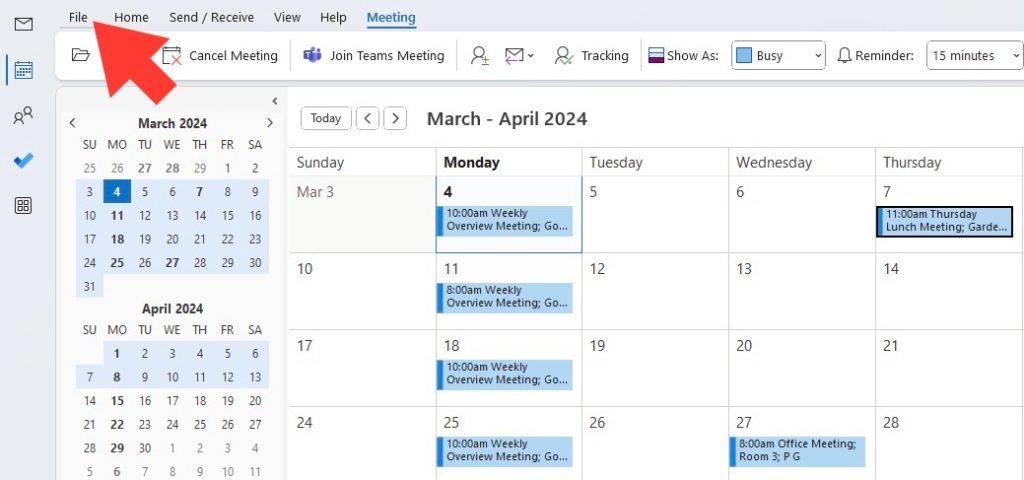The image showcases a Microsoft Calendar display with several notable features. A prominently added large red arrow, angled in the northwest direction, is pointing at the "File" menu at the top of the calendar interface. The interface's top section includes a gray navigation bar featuring options such as File, Home, Send/Receive, View, Help, and Meeting. Notably, "Meeting" is currently selected, highlighted in blue text with a blue underline.

Beneath this navigation bar, additional meeting-related options are visible, though partially obscured by the red arrow. These options include icons and commands for canceling a meeting (featuring a calendar with a red X), joining a Teams meeting (indicated by the Teams icon), adding participants (represented by a portrait icon with a plus/minus sign), and sending messages (an arrow pointing left). Further options include a participant tracker (person icon with a green check), status modification (currently showing "Busy" with a blue square), and a reminder setting (bell icon with a dropdown indicating 15 minutes).

The primary view is the calendar for March and April 2024, arranged in a grid format. Days of the week from Sunday to Thursday are visible, with the rest cut off. Notably, Mondays are bolded, particularly Monday, March 4th, highlighted indicating the selected date. Calendar events include a recurring "10 a.m. Weekly Overview Meeting" on all Mondays, a "Thursday Lunch Meeting, Garden" at 11 a.m. on March 7th, and an "8 a.m. Office Meeting, Room 3 PG" on Wednesday, March 27th.

To the left, miniature calendar views for both March and April 2024 are displayed. Highlighted regions in light blue span from Sunday, March 3rd to Sunday, April 7th on the left segment, and Saturday, April 13th on the right segment, with the selected date marked by a dark blue box around the numeral 4 for Monday, March 4th.

The leftmost side of the screen houses a simple navigation bar featuring a selected keyboard icon marked by a blue vertical line. Beneath it are icons depicting two people, a blue checkmark with a blue square tip, and a grid of four squares. The remainder of this navigation bar is empty.